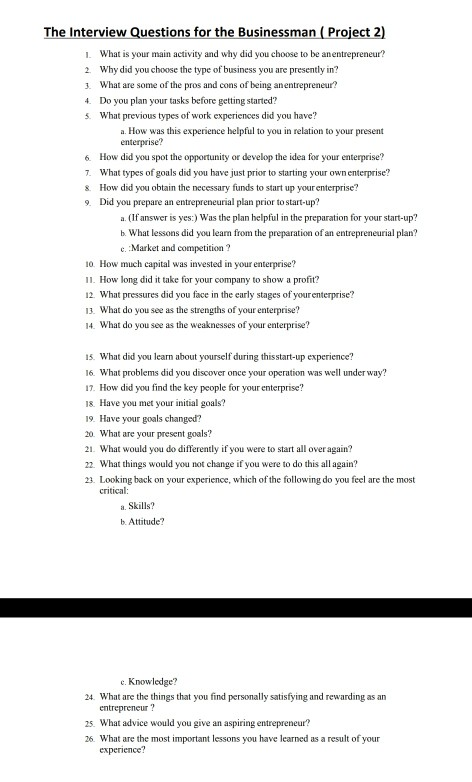This image features a comprehensive list of 26 interview questions designed for a businessman, labeled as "Interview Questions for the Businessman (Project Two)." The questionnaire aims to delve deeply into the experiences and insights of an entrepreneur. Here’s an overview of some of the key questions:

1. **Main Activity and Choice of Entrepreneurship:** The first question asks about the primary business activity and the motivation behind choosing to be an entrepreneur.
2. **Type of Business:** The second question probes into why the businessman chose his specific line of business.
3. **Pros and Cons:** The third question seeks to understand the advantages and disadvantages of being an entrepreneur.
4. **Task Planning:** The fourth question inquires if the entrepreneur plans tasks before initiating them.
5. **Work Experience:** The fifth question, along with a sub-question, asks about previous work experiences and how they have been beneficial in the current business.

Skipping to later questions:
18. **Initial Goals:** Asks if the entrepreneur has met their initial goals.
19. **Goal Evolution:** Inquires whether the goals have changed over time.
20. **Present Goals:** Asks about the current objectives.
21. **Retrospective Changes:** Questions what the businessman would do differently if starting over.
   
Following a black box that appears to indicate a page change:
24. **Personal Satisfaction:** Asks what aspects of entrepreneurship the businessman finds satisfying and rewarding.
25. **Advice for Aspiring Entrepreneurs:** Seeks advice for those looking to start their own ventures.
26. **Important Lessons:** Inquires about the most important lessons learned from the entrepreneurial journey.

This detailed list appears designed to extract valuable insights, experiences, and advice from seasoned entrepreneurs.